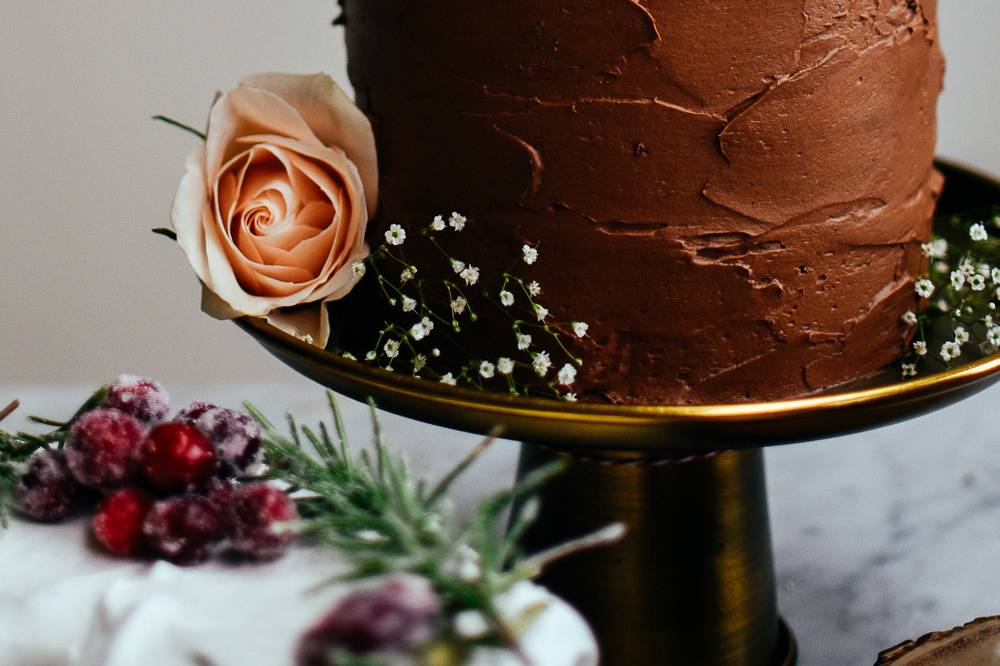This is a refined and detailed caption merging the descriptions provided:

The image features a decadent chocolate cake, prominently displayed on an elegant, shiny gold or brass cake platter that is elevated above a table. The cake itself is adorned with chocolate frosting, applied in a messy, unsmooth manner, giving it a homemade charm. To the left of the cake, a peach or light pink rose adds a touch of romance, while small white flowers delicately decorate the mid-left and far-right sides of the platter. On the table alongside the cake, there's another pastry, seemingly covered in white frosting with a hint of red berries, possibly cherries or frozen cranberries, and pine needles, enhancing the festive atmosphere. The background fades into a soft blur, highlighting the cake and floral decorations in sharp focus. The overall composition is classy and elegant, suggestive of a sophisticated wedding setting and captured in a contemporary, high-quality stock photo style.